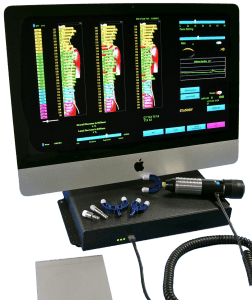The image depicts an Apple computer monitor with an integrated CPU, placed on a black electronic base. The monitor, identifiable by the Apple logo on a silver strip at the bottom, displays a dark background with vibrant graphical elements including red, yellow, green, blue, and purple vertical lines, which appear to be data analysis graphs. The screen also features additional graphics and buttons on the right, possibly for further data interaction, although the written content is indecipherable. Below the monitor is a black box, which has several cords and cables attached, including a coiled one, and three green LEDs on its surface. This box might be connected to a handheld measuring instrument, potentially for thermal or electrical analysis, given the presence of various white and blue tips nearby that could be affixed to the device. The overall setup suggests a sophisticated data evaluation or monitoring system.